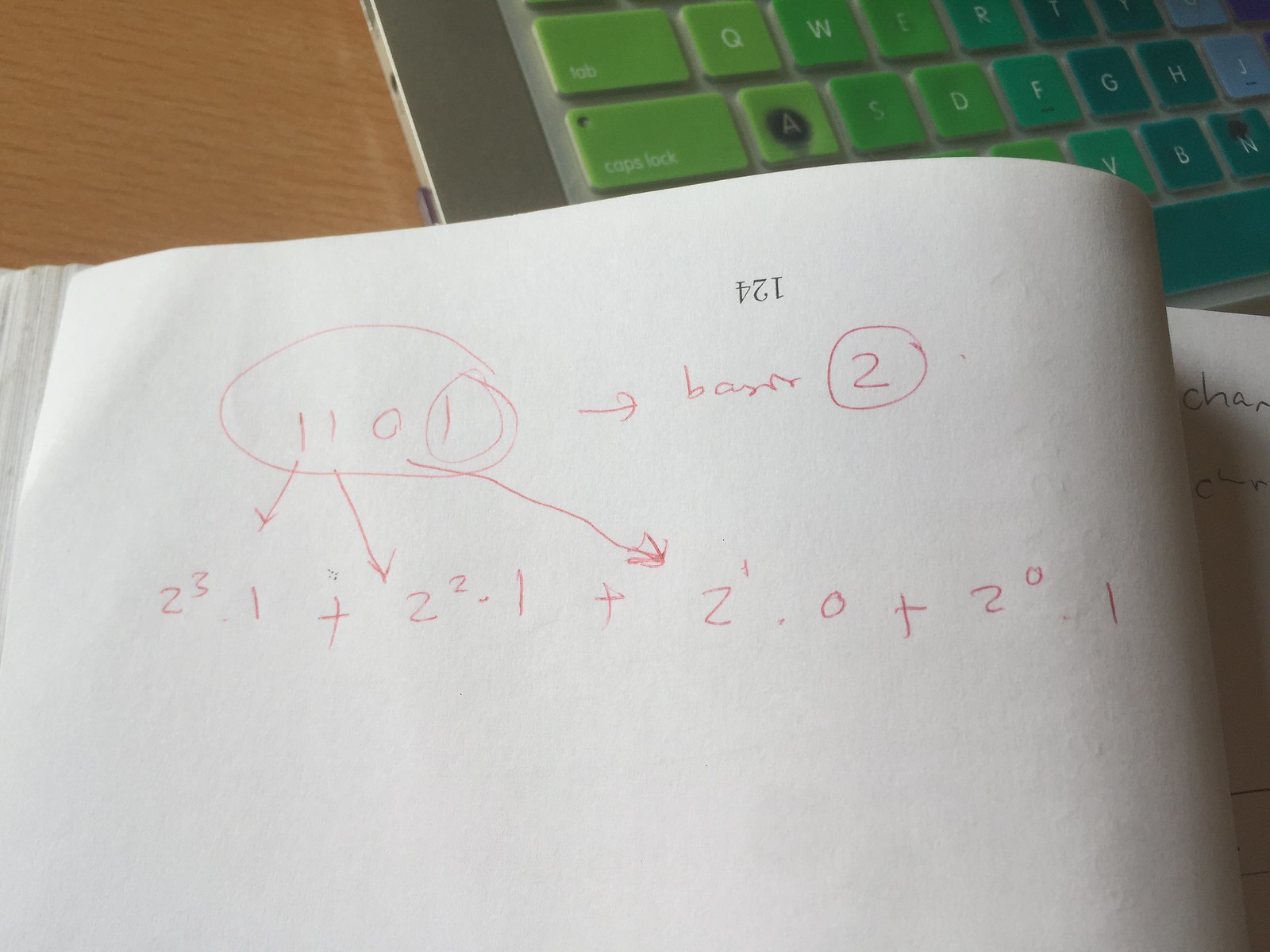In the image, a silver laptop with a prominently visible left border is positioned on a medium-light wood table, possibly made of linoleum mimicking wood. The laptop's keyboard features an interesting color gradient, beginning with light green keys including the Tab, Caps Lock, Q, and a worn A key, showing signs of heavy use with black marks in a circular pattern. As you move rightward across the keyboard, the keys transition through shades of medium green to aquamarine, then to dark blue at the center, and finally to a light blue with a hint of purple.

In front of the laptop, an upside-down book, likely a sketchbook or a math book, is open, revealing a page filled with handwritten equations. The page features a black printed number "124" in the upper middle area, oriented upside down. Additionally, there is red handwriting that includes the number "1101," with the first "1" circled and the entire equation circled in an oval. Various arrows and annotations adorn the page, including markings such as "2^3" (two to the third power), "1 +", with arrows from "1" pointing to "2", followed by a question mark, "1 + 2", and another arrow from "0" pointing to "2^1", then "0 + 2^0 + 1".